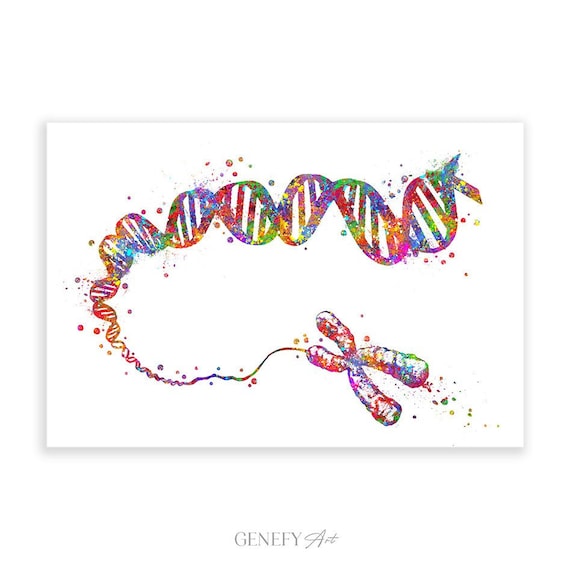The image showcases vibrant, celebratory artwork on a white background. Dominating the piece is a DNA double helix and an X chromosome, both depicted in bold, rainbow colors. The DNA strand is oriented diagonally, rotated counterclockwise, extending from the lower right to the upper left. This helix intertwines seamlessly with the X chromosome positioned in the image's upper right corner. Radiating dots of various sizes surround these elements, adding a sparkly, playful atmosphere. The DNA strand becomes wider as it ascends, culminating in slightly unfurling strands at the top. Below the image, the text "GENIFY ART" is prominently displayed, with "GENIFY" in all capitals and a serif font, while "art" is written in a more whimsical, cursive style. This piece exudes a lively and engaging aesthetic, suitable for display in settings such as a doctor's office.